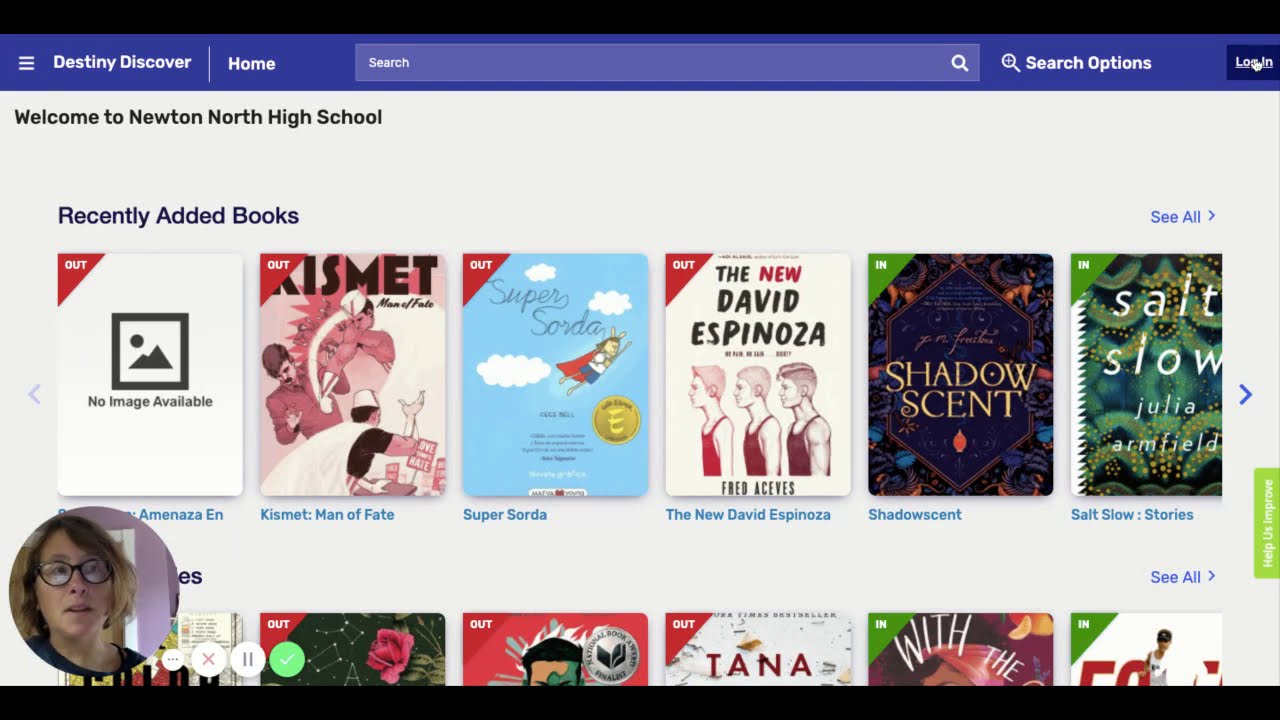The image is a screenshot of a graphical user interface from a library application, likely associated with Newton North High School. The interface resembles a typical computer screen layout with a purple horizontal menu bar at the top, featuring white text that reads "Destiny Discover," followed by various navigation options like "Home" and a search bar with search options, and a "Login" button. Beneath the menu bar, the main section of the page is prominently divided into different sections showcasing rectangular book covers. The highlighted section is titled "Recently Added Books," displaying a row of six books: the titles include "Kismet," "Super Sorta," "The New David Espinosa," "Shadow Scent," and "Salt Low," with one book not showing an image. The availability status of the books is indicated by green "In" or red "Out" labels in the upper left-hand corners of the book images.

Additionally, there is a small, circular webcam feed in the bottom left-hand corner, featuring a close-up photo of a woman. Surrounding the webcam photo are small icons for actions like "Pause," "X," and "Checkmark." The background of the web page includes a blue border and a light blue backdrop, which frames the content neatly. The content beneath the recently added books appears partially obscured by the webcam feed, making it difficult to see additional book lists or details.